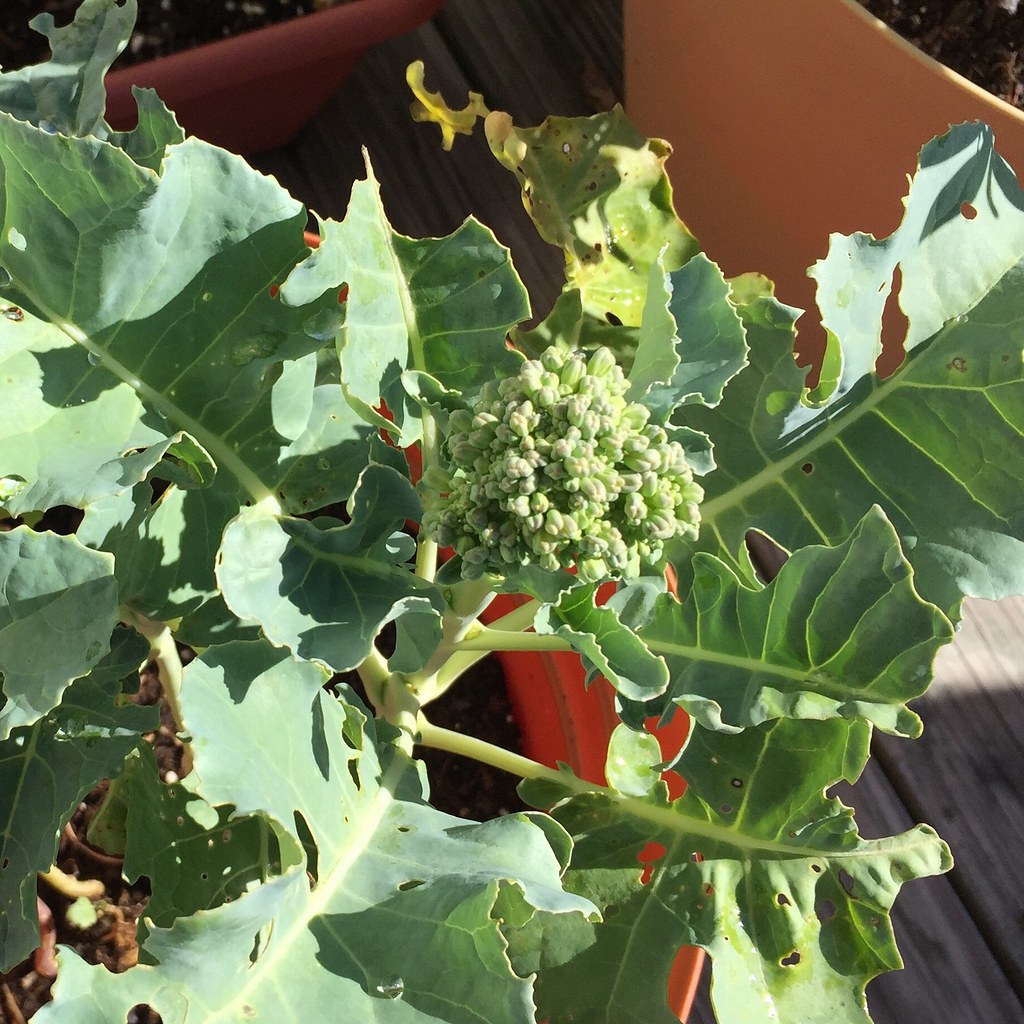This color photograph, taken in daylight, features a close-up, top-down view of a plant growing in a large orange pot sitting on a wooden deck. The plant, which resembles a young edible vegetable like broccoli, broccolini, or cauliflower, has thick, dark green leaves with detailed ribbing and veins that give a textured appearance. The leaves display signs of being eaten by bugs, resulting in jagged edges. At the plant's center, there's an immature head or cluster of light green buds. Surrounding the plant and pot, you can see sections of old wooden planks and the outlines of additional terracotta pots in the background, alongside cardboard boxes catching the sunlight. The photograph captures the interplay of light and shadow, highlighting the plant's details and the rustic setting.